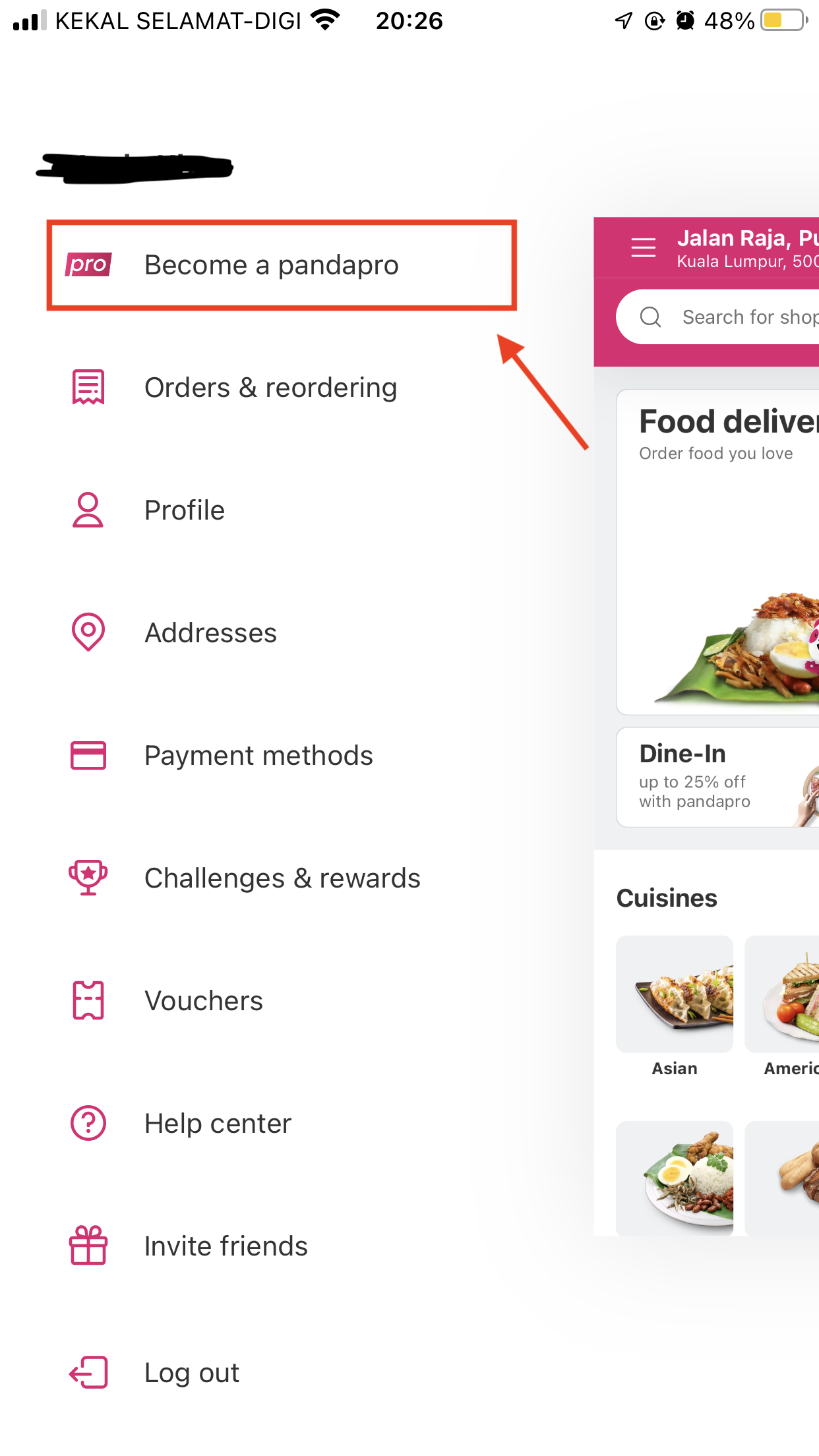The top left corner of the image displays the signal strength icon, followed by the Wi-Fi status and the current time, which is shown as 20:26. On the right-hand side, a series of icons are visible, including an alarm clock and a battery indicator displaying 48% with a yellow gauge.

Below this status bar, the screen appears to show a settings page for a website. Prominently featured at the top is a heading labeled "Become a PandaPro," highlighted with a red square and indicated by a red arrow. Underneath this are headings like "Orders and Reordering," "Profile," "Addresses," "Payment Methods," "Challenges and Rewards," "Vouchers," "Help Center," "Invite Friends," and "Log Out." Each of these items is accompanied by a simple pink icon on the left, symbolizing its respective category. 

On the right side of the screen, there are elements that suggest details of a food delivery service, including options for dining in or takeaway. Photographs of different cuisines, such as Asian and American food, are displayed, providing a visual guide to the menu offerings.